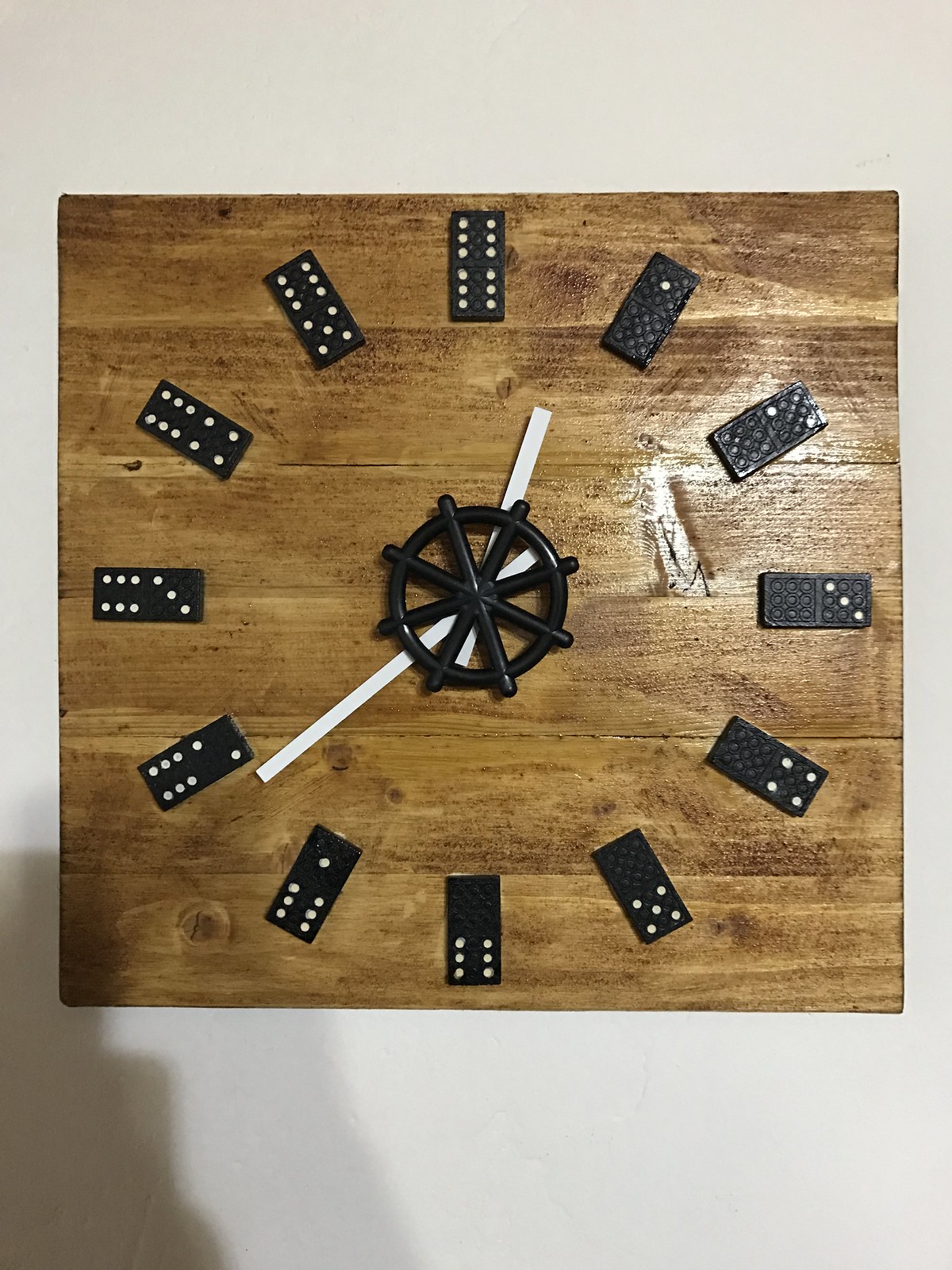A uniquely crafted clock face made entirely from dominoes is mounted on a wooden surface that is affixed to a wall. Each hour is marked by a specific domino: the double six domino represents twelve o'clock, the zero-one for one o'clock, the zero-two for two o'clock, and so forth, continuing in this pattern until the five-six domino, which designates eleven o'clock. At the center of the clock, there's a black circular element with radial lines resembling a wagon wheel, through which the white hour and minute hands are visible. The hour hand is positioned just before the one, indicating it's almost one o'clock, while the minute hand is approaching the eight, suggesting a time close to 12:40. The wooden backdrop enhances the artistic and rustic appearance of this unconventional timepiece.